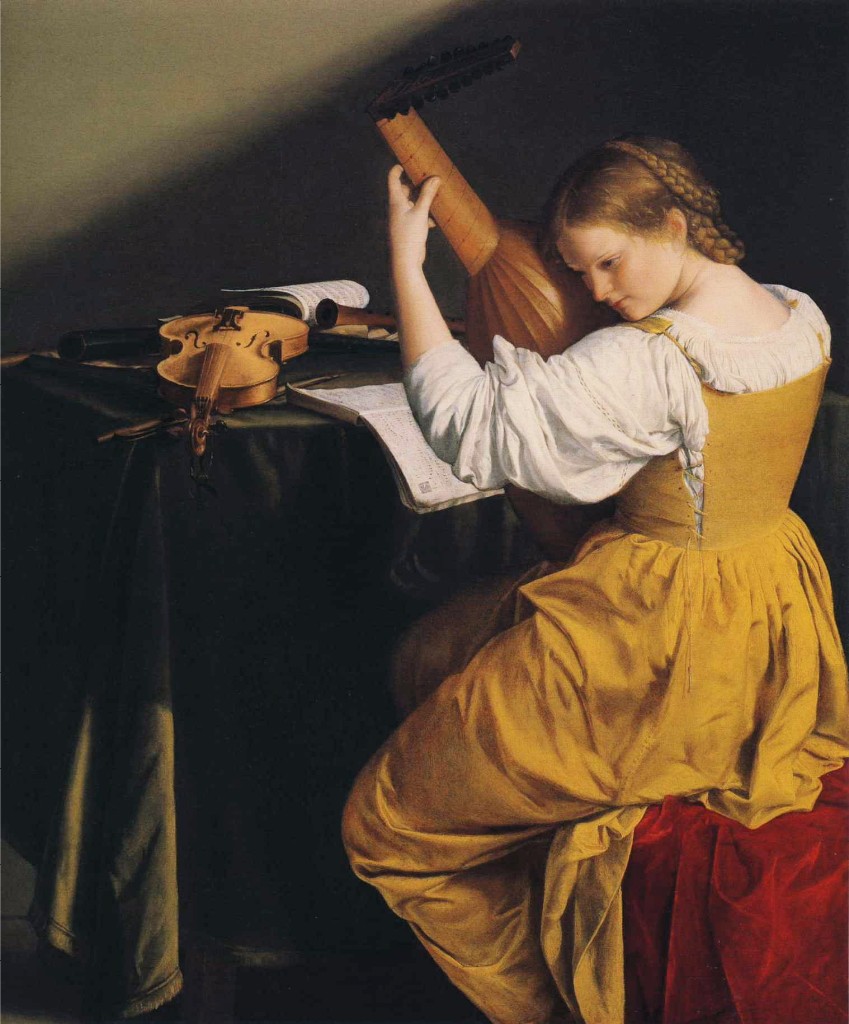The painting depicts a woman in a yellow dress with a white puffy blouse, her light brown hair styled in braids wrapped around the back of her head. She sits on a red velvet stool, positioned in the right third of the canvas, in front of a table draped in green velvet. The woman gazes downward and to her left as she cradles a stringed instrument, about the size of a small guitar, with its neck bent and the strings out of view. On the table before her lies an assortment of items, including a violin or viola with a bow beneath it, sheet music, and potentially a wind instrument. The backdrop is mostly dark, with a touch of olive green in the top left corner, lending a rich, somewhat somber atmosphere to the detailed, European-style scene, reminiscent of the 16th or 17th century.